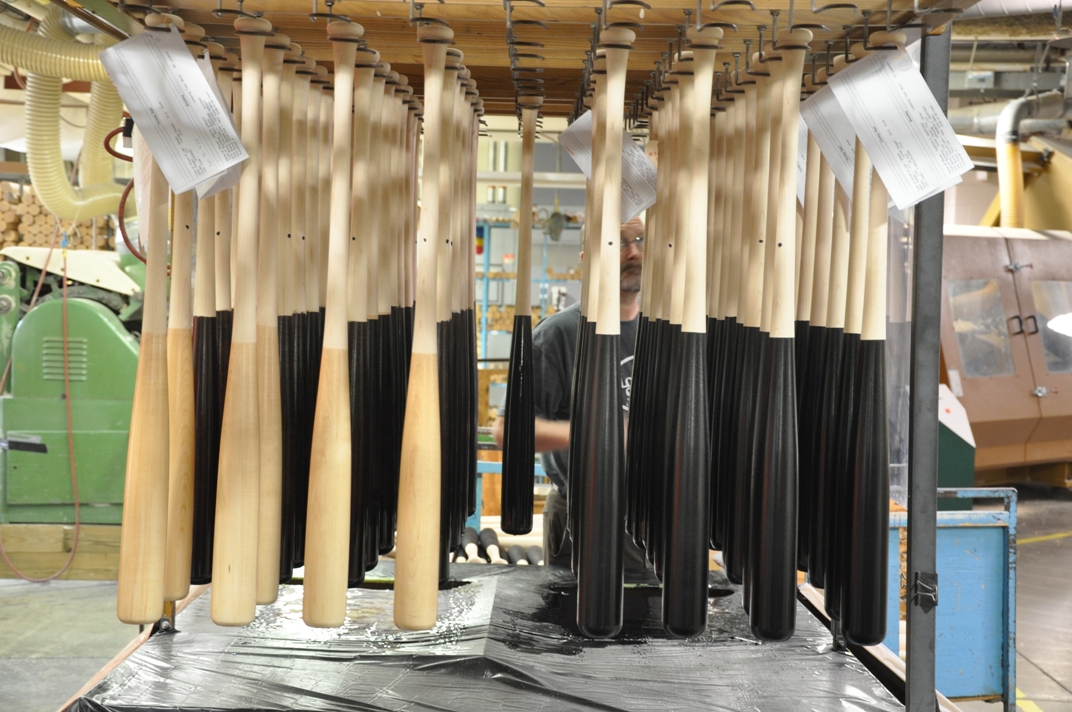The image depicts a production plant, specifically a factory assembly line dedicated to manufacturing wooden baseball bats. Central to the image is a metal stand equipped with hooks from which dozens of baseball bats hang in neat, organized rows, forming a square pattern. The bats are suspended upside down, with their handles secured in metal rings. Many of the bats feature a dual-tone design: the handles are left with a light wood grain finish, while the barrels are painted black. A few bats retain a uniform light tan color, perhaps indicating a different stage in the finishing process. 

In the background, the factory setting is highlighted by an array of industrial equipment and wooden materials. Visible items include a brown piece of machinery with windowed doors and handles, a blue metal cart, and a partially obscured green heavy machine. Stacks of wood are piled up in the left part of the backdrop, hinting at the raw materials used in the bat production. A tarp with paint marks lies beneath the bats, suggesting recent painting activity. Additionally, several bats have pieces of paper attached to their handles, likely containing production details.

A man dressed in a black shirt, apron, and glasses can be seen inspecting the bats, indicating an ongoing quality check or completion of the manufacturing process. The presence of tubes and venting systems further emphasizes the industrial nature of the setting. Overall, the image captures the detailed and organized environment of a baseball bat production line in full operation.